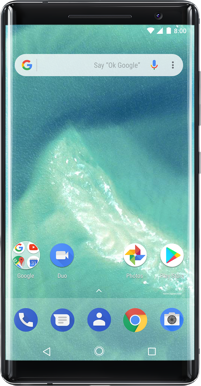The image depicts a smartphone screen with a noticeable black outline. At the top of the screen, a search bar stretches from the left to the right side. In the left corner of the search bar, the distinctive Google "G" logo is present, which is red at the top, yellow on the right, green at the bottom, and blue on the left. Inside this search bar, the text "Say 'OK Google'" appears in black with "OK Google" in quotations. To the right of this text is a microphone icon illustrated in Google's signature colors: blue, yellow, red, and green. Further to the right, there are three vertically aligned black dots.

The wallpaper on the phone displays a striking image of ocean water, characterized by its bluish-green hue. Emerging from the bottom right-hand corner and almost diagonally upward is a splash of red within the water.

Near the bottom of the screen, various icons are organized. Starting from the left, there is a bar hosting four icons in white circles. The first icon is the multicolored Google logo. Next to it lies a white circle containing the YouTube logo with a red box. Below this is an icon resembling Google Maps. Adjacent is another white circle featuring a blue box and the text "Google" in white underneath. To the right, a blue circle with a white video camera icon is labeled "Duo" in white text below.

Beyond a small gap, on the far right side, a white circle encompasses an icon that resembles a fan, with yellow and green on the left side, and red and blue on the right side. Below it is the label "Photos." Another white circle within this row contains the Google Play logo in red, yellow, green, and blue. However, the text beneath this logo is somewhat obscured by the wallpaper's white tones and is illegible.

Beneath this row lies another set of icons. This row starts with a blue circle housing a white phone icon, followed by a blue circle with a white piece of paper. Next in line is a blue circle displaying a white icon of a person. Beside it sits the distinctive Google G-ball, featuring segments in red (top), green (side), yellow (left), and blue (center). Another blue circle with a white phone icon is present, followed by a white arrow pointing left, a white circle, and finally a white square at the bottom of the screen.